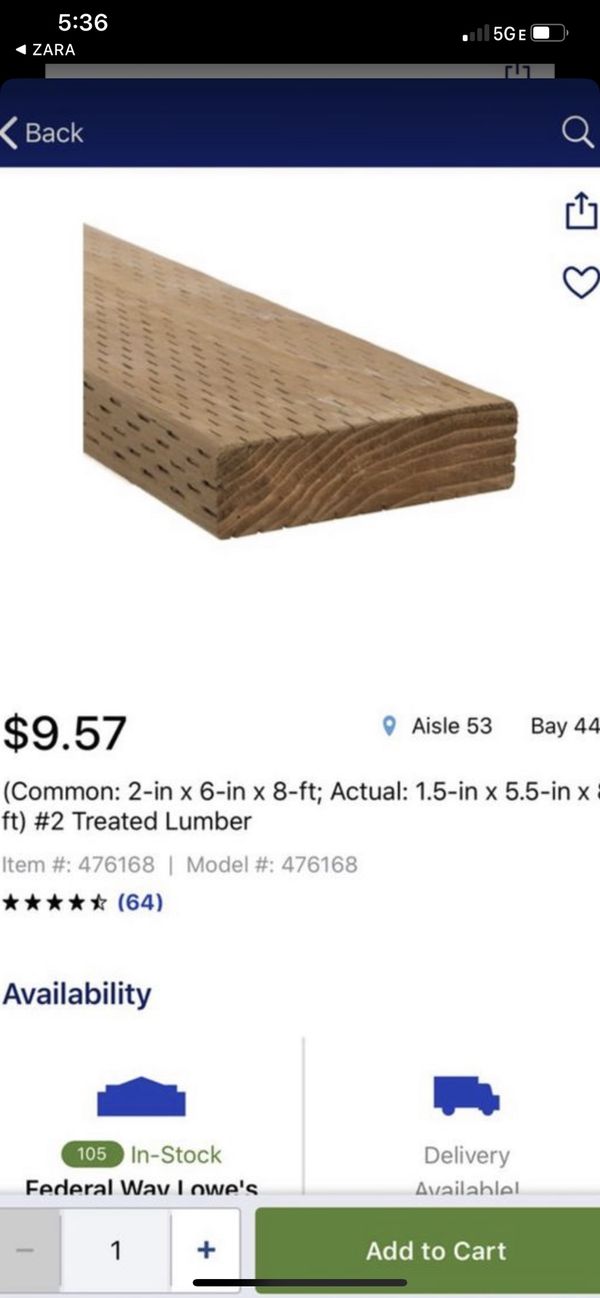This detailed description highlights various elements seen in a screenshot from a shopping website:

*The top portion of the screenshot features a black background spanning about half an inch. In the top left corner, the number "536" is displayed, with a small white triangle pointing leftward underneath it. Adjacent to the number, the word "Zara" is positioned prominently. On the right side, a partially full battery icon reads "5G E" and indicates one out of four available internet bars.*

*Beneath this section, a thin gray border extends approximately a quarter inch from both the left and right edges. Moving further down, there is a half-inch blue border on the left side, marked by a gray greater-than symbol pointing left. Additionally, a gray search icon is located on the right side.*

*The main content area features a white background. Around the midway point, the image captures the end of a piece of wood pointed down and to the right. In the top right corner, there's a download icon and a blue heart icon with a white interior below it.*

*Towards the lower left section, the number "957" is indicatively marked, stating its position on aisle 53 by 54. Below this, detailed information about the lumber is provided including the item and model numbers, star rating, and availability status in blue text. A blue building icon represents its onsite availability at the location mentioned.* 

*Alongside this, the words "Industry in Stock Federal Raise Federal Weigh Lows" appear, divided by a vertical line next to a blue truck icon that states "Delivery Available."*

*At the bottom, there is a gray search rectangle with a black square on the left side followed by a gray square containing a gray minus sign. Next to it, a white square with a black numeral "1" is positioned beside another gray square featuring a blue plus sign. This section culminates with a large green button labeled “Add to Cart” in white text.*